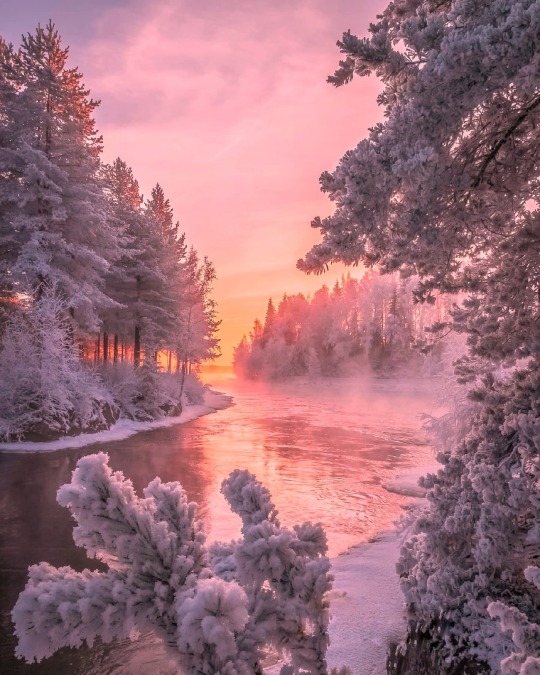This captivating photograph captures a serene winter forest scene at sunset, with a gentle, meandering river flowing through it. The banks of the river and the ground are partially covered in snow and ice, indicating the tail end of winter. Pine trees on both sides, laden with melting snow, add to the enchanting atmosphere. The muting of the snow creates visible definitions on the branches of the dark green evergreen trees that stretch across the landscape. The sky at the horizon glows with a warm, fiery orange hue, transitioning into shades of pink and purple, which are beautifully reflected in the river’s calm surface. A soft mist rolls over the water, enhancing the dreamlike quality of the image. The fading light casts a glow on the frozen landscape, giving the scene a magical, almost otherworldly appearance.